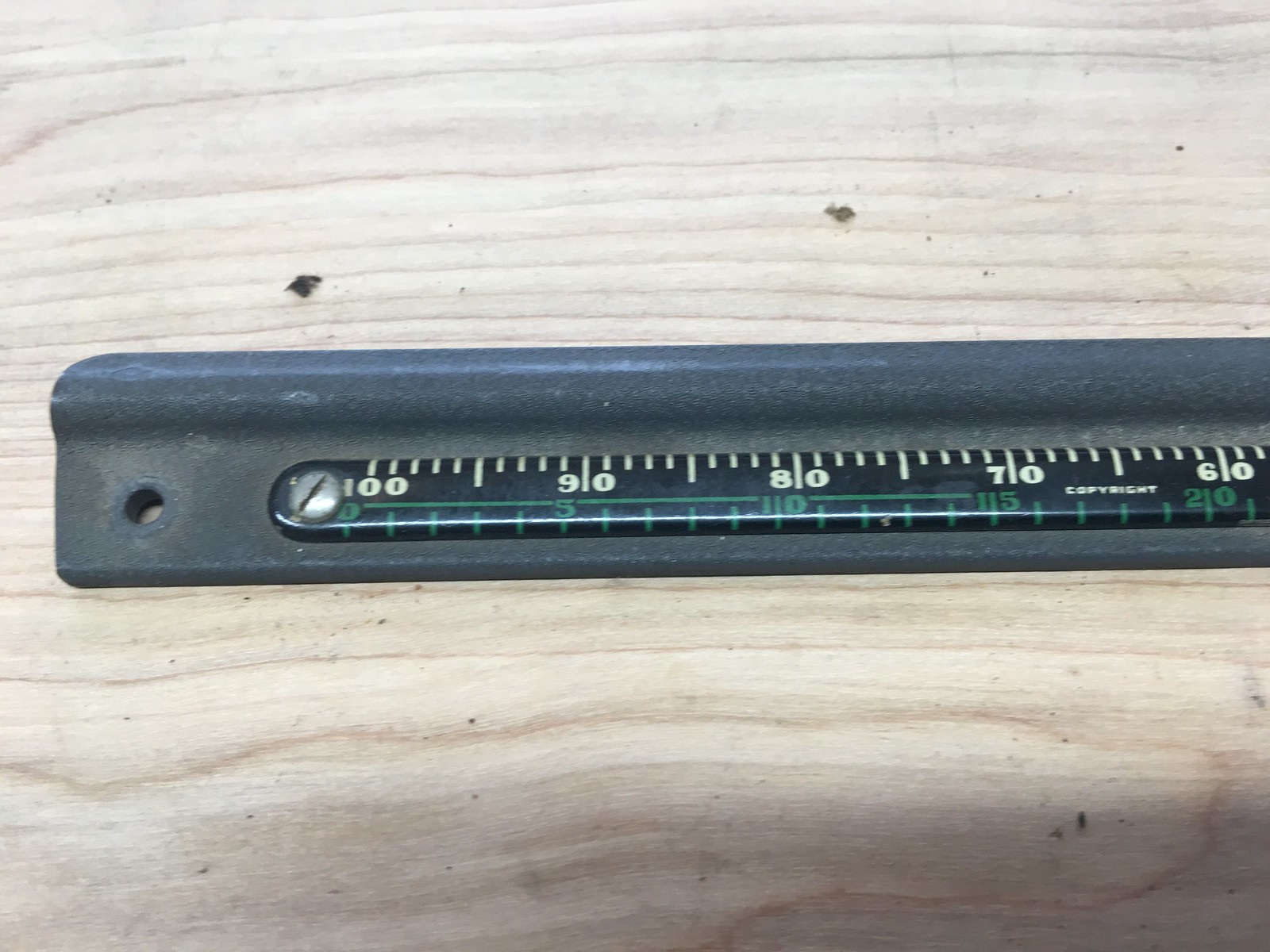The image features a black roller gauge placed against a light-colored wooden table. The roller gauge is marked with measurements, possibly in millimeters and inches, with the top markings reading 100, 90, 80, 70, and 60, and the bottom markings reading 0, 5, 10, 15, and 20. A steel metal screw is positioned on the left side, partially obscuring the numbers 0, 1, and 100 on the roller. The background wall is also made of wood, featuring vertical lines, a nail, and a screw on the left side. The table below the roller has some black specks scattered at the top left and middle right sections. There is a noticeable shadow at the bottom of the image, and some plastic bits are visible on the table.